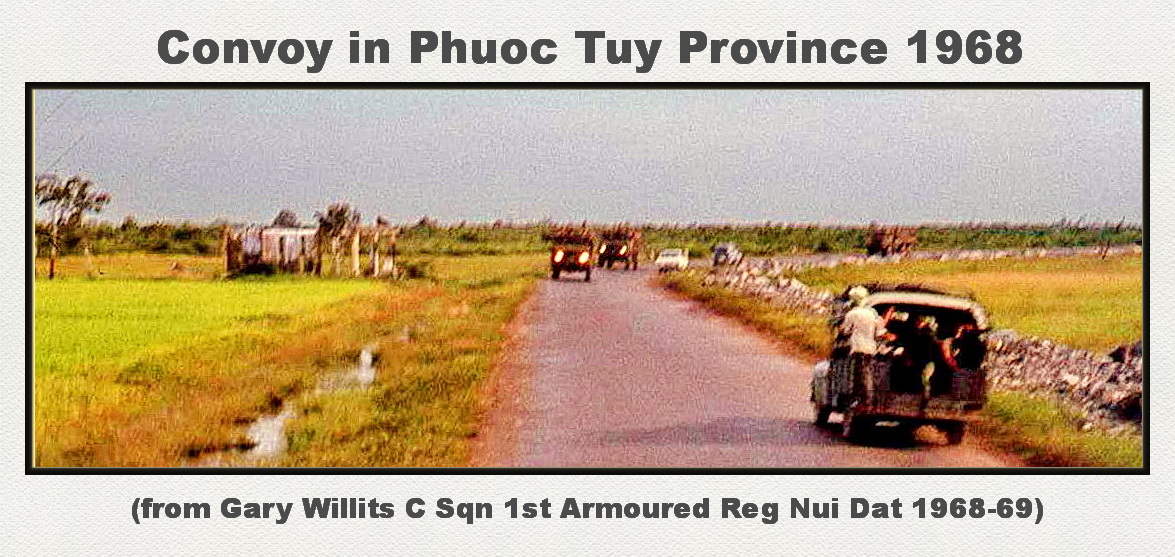This colored, yet slightly blurry, photograph from 1968 shows a convoy scene set in Phuoc Tuy Province. Central to the image is a dirt road originating from the bottom right and extending into the center, where it sharply turns to the right. The road is flanked by green grasslands, appearing somewhat marshy, and has a brown hue with cobblestone fencing visible on the right-hand side. On the road, a truck with an open back can be seen heading away, carrying a couple of people, while two approaching trucks, possibly military-grade, advance alongside smaller vehicles with their headlights gleaming. The setting includes a few scattered trees and an old derelict building off to the left, contributing to the barren landscape. Above the image, the caption reads "Convoy in Phuoc Tuy Province, 1968," and below it notes, "From Gary Willett, C. Sqn, 1st Armored Regiment, Nui Dat, 1968-1969."